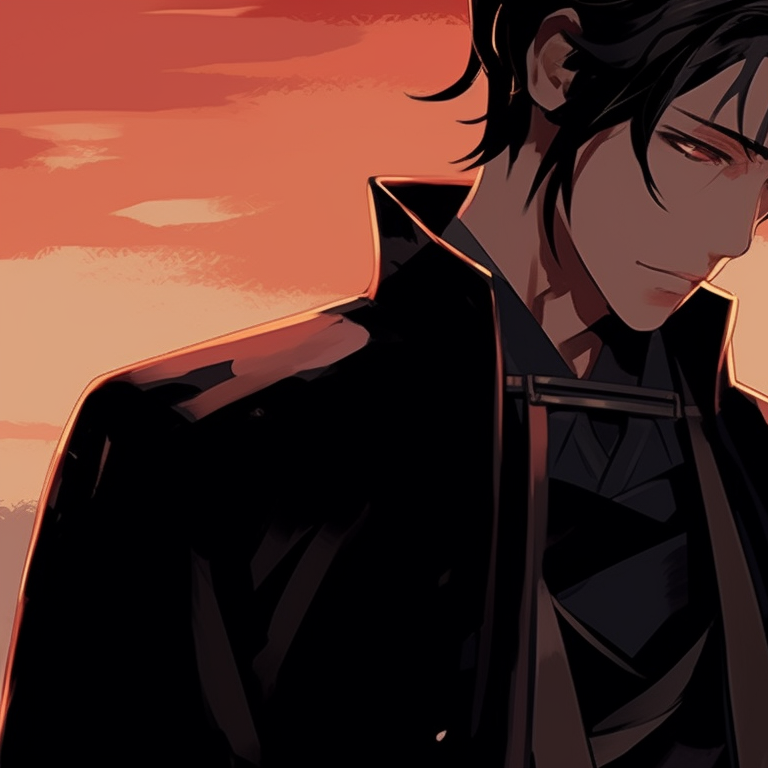This image depicts a melancholic anime male character with white skin, staring downwards to the right. His chiseled face is framed by short, tousled black hair that falls into his face, partially obscuring his thin black eyebrows and striking yellow eyes, which contribute to his sorrowful expression. He is attired in a dark, futuristic ensemble, featuring a black cloak fastened with a unique iron clasp at the neck and a matching black shirt underneath. Illuminated by the warm, golden hour light, the backdrop consists of a vivid sunset sky with hues of orange, pink, and red that reflect off his jacket, enhancing the overall somber mood of the scene. The square-shaped image captures a poignant and simple setting, further emphasizing the character's deep sense of sadness.